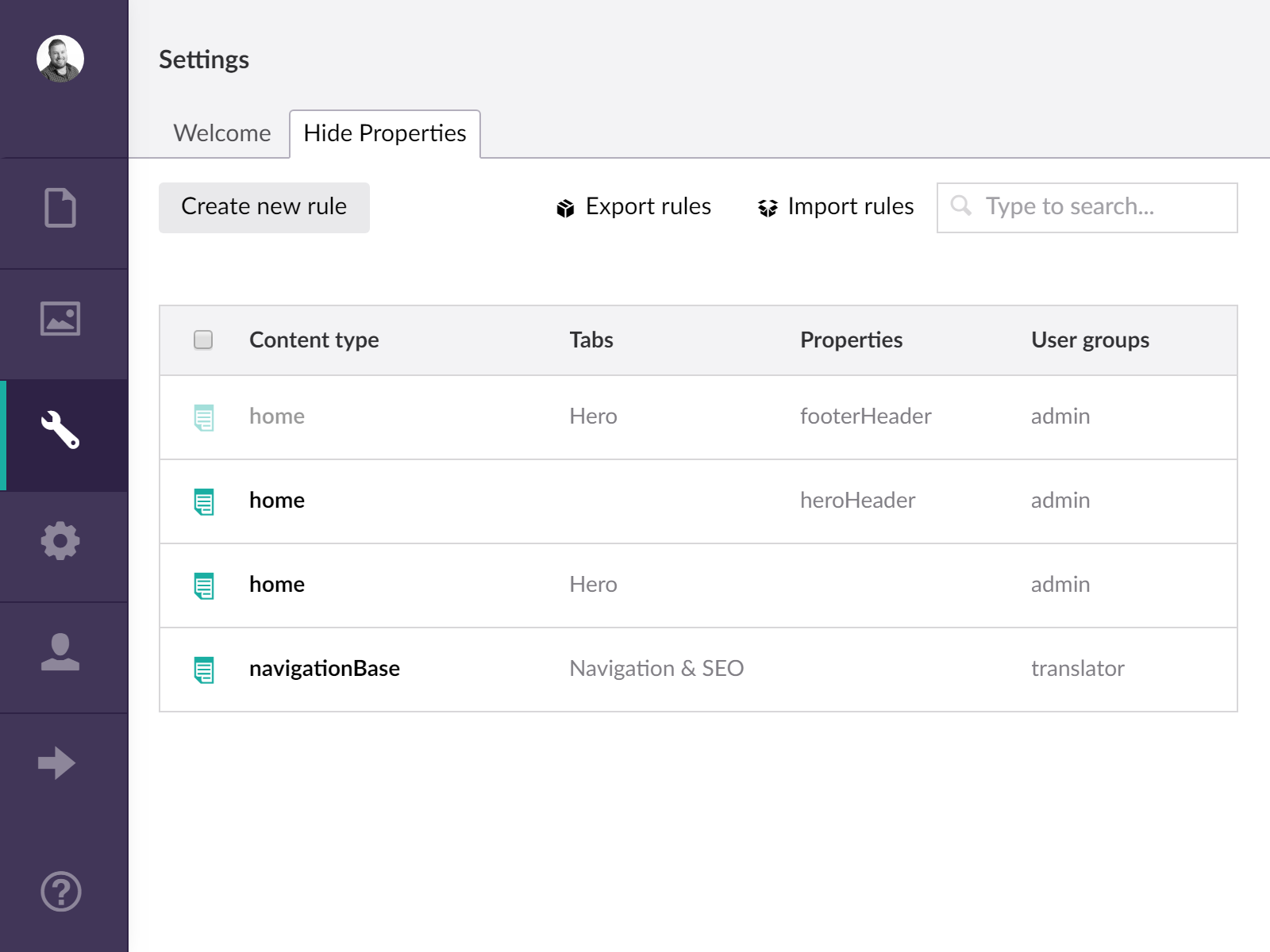This is a detailed screenshot of a web application interface. The interface features a prominently displayed purple sidebar on the left side of the screen, housing several navigation tabs. At the very top left, there is a monochromatic black and white profile picture of a smiling gentleman, enclosed within a circular bubble. 

The sidebar includes six distinct tabs, each represented by an icon:
1. The top icon is an image of a page.
2. The second is a gallery image.
3. The third, currently highlighted, is a wrench, indicating the current tab.
4. The fourth is a cogwheel, likely representing settings.
5. The fifth is an image of a human silhouette, presumably for the profile page.
6. The last icon is a right-pointing arrow, likely functioning as a sign-out button.

Additionally, there is a question mark icon at the bottom left corner, typically used for help or support.

The main area of this page displays the "Settings" section, which is divided into two tabs: a "Welcome" tab and a "Hide Properties" tab. The "Hide Properties" tab is currently active. Within this active tab, there are several functionalities available, including buttons labeled "Create New Rule," "Export Rules," and "Import Rules." A search box is also present for easy filtering.

Moreover, various sections such as "Home," "Navigation Base," "Different Tabs," "Properties," and "User Groups" are listed. Under "User Groups," three groups are labeled as admin, and one is identified as a translator.